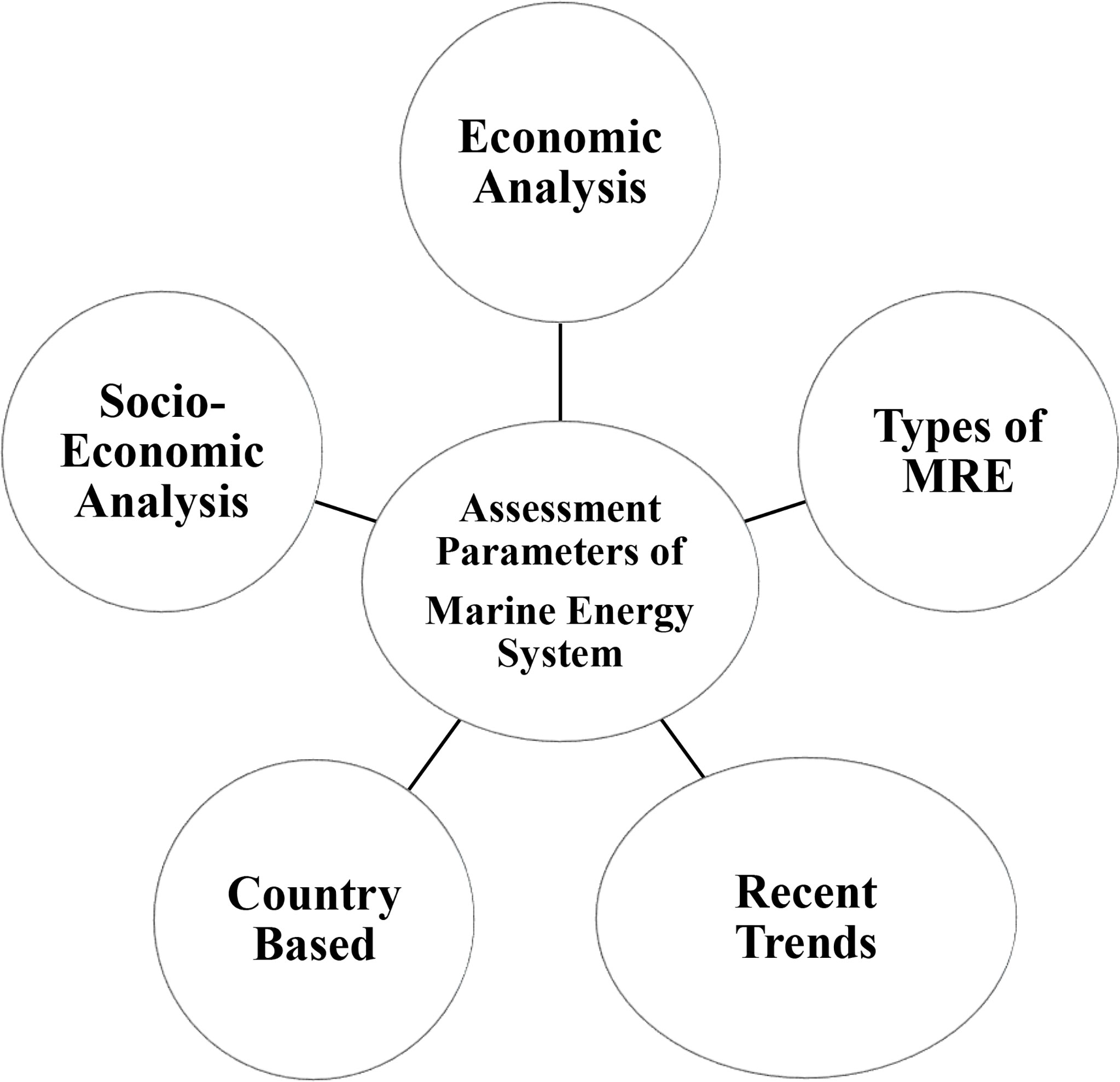The image is a black-and-white bubble diagram featuring a central circle labeled "Assessment Parameters of Marine Energy Systems." Surrounding this central circle are five smaller circles, each connected to it by lines. The top circle is labeled "Economic Analysis"; the right circle reads "Types of MRE"; the bottom right circle says "Recent Trends"; the bottom left circle is labeled "Country-Based"; and the left circle reads "Socioeconomic Analysis." Each circle is outlined in a grayish-black trim and contains black font text. There are no large bold letters, and the font size appears fairly uniform across all labels. The background of the image is plain white, with no additional colors or graphical elements.